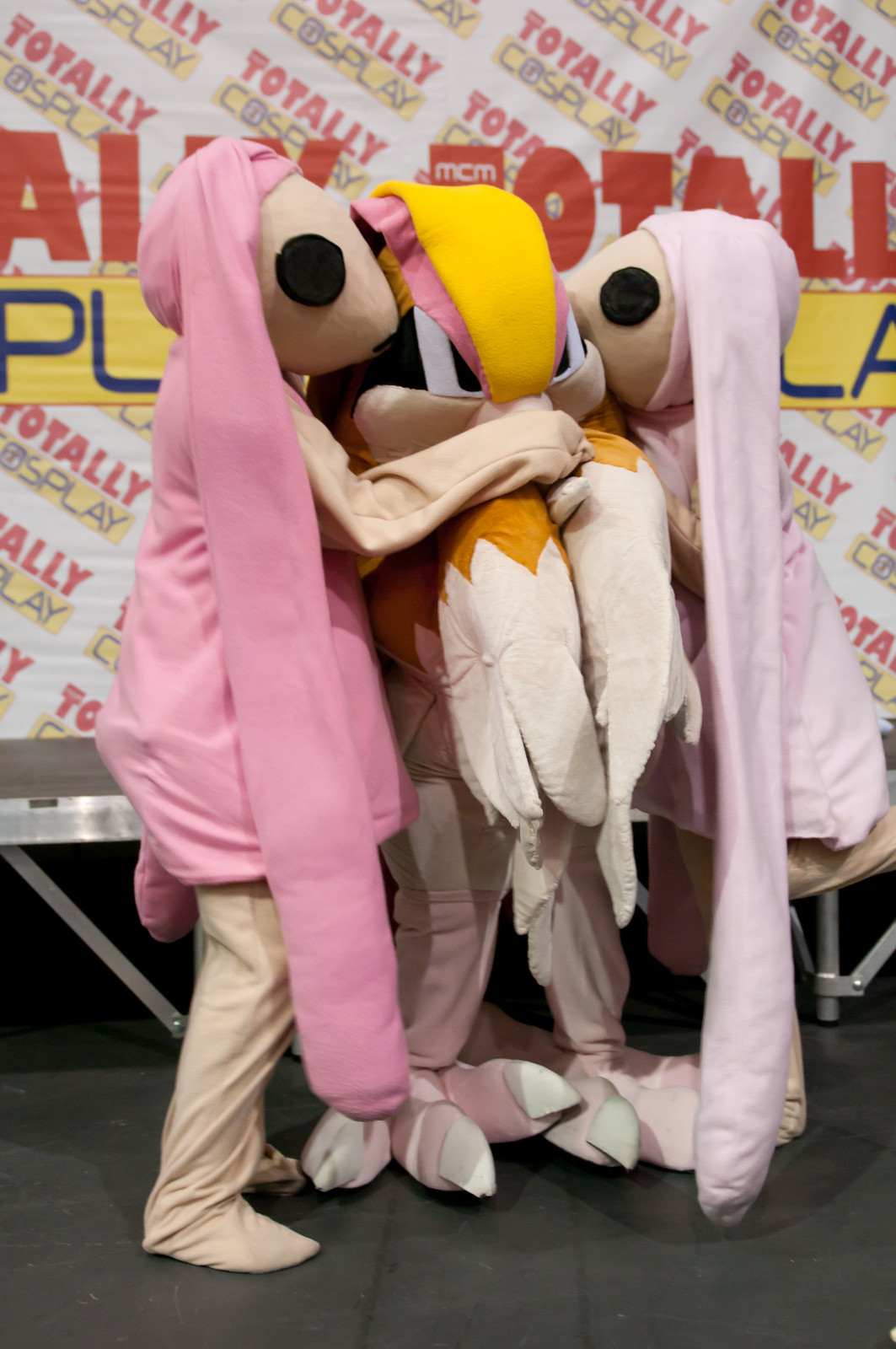The image captures a vibrant scene at a cosplay event, as indicated by the recurring text "TOTALLY COSPLAY" in bold red and blue lettering against a yellow background. The central figure is dressed as Lola Bunny from Space Jam, with distinctive features that blend dinosaur or bird-like qualities—most notably, her feet which are adorned with claws or talons. Flanking her are two other cosplayers who share a similar theme. They both don pink hats, which resemble whimsical capes or hoods—one in bright pink and the other in a lighter shade. Each wears a white outfit with matching pants and sport black button eyes, which add a playful, cartoonish touch to their appearance. The cosplayer on the left has a pink shirt, while the one on the right is facing the opposite direction in a lighter pink shirt and prominent ears or headgear. The middle cosplayer's costume is detailed with a yellow head covering, pink accents, white and orange wings, and a black base, completing the ensemble with white toenails or talons. The group poses joyfully amidst the backdrop, suggesting they've come together specifically for this engaging and colorful cosplay event.